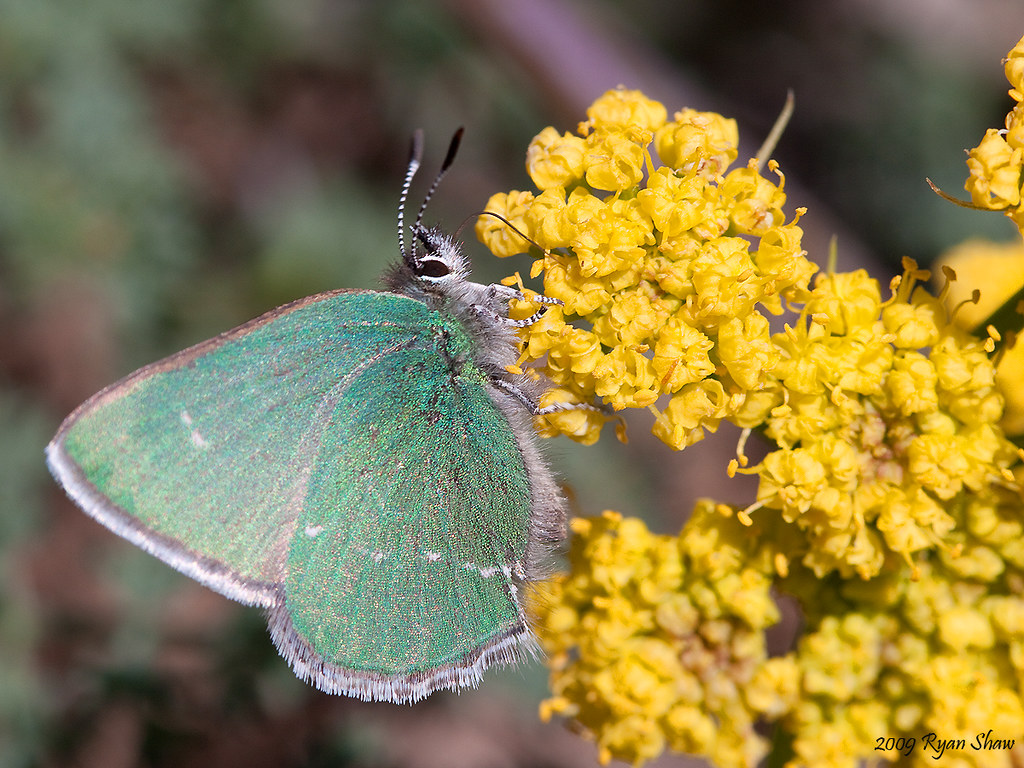This detailed image captures a vibrant scene of a butterfly pollinating yellow flowers. The butterfly, with its furry gray body and striking shimmery emerald wings bordered by delicate gray hairs, is perched at an angle on a cluster of small, round yellow flower pods that resemble popcorn. Zoomed in for close detail, the photo highlights the butterfly's big black eyes and long, gray and black antennae. The background, a mix of blurred green and brown hues, subtly frames this lively interaction with nature. In the bottom right-hand corner, the photo is marked with the text "2009, Ryan Shaw," indicating its copyright.